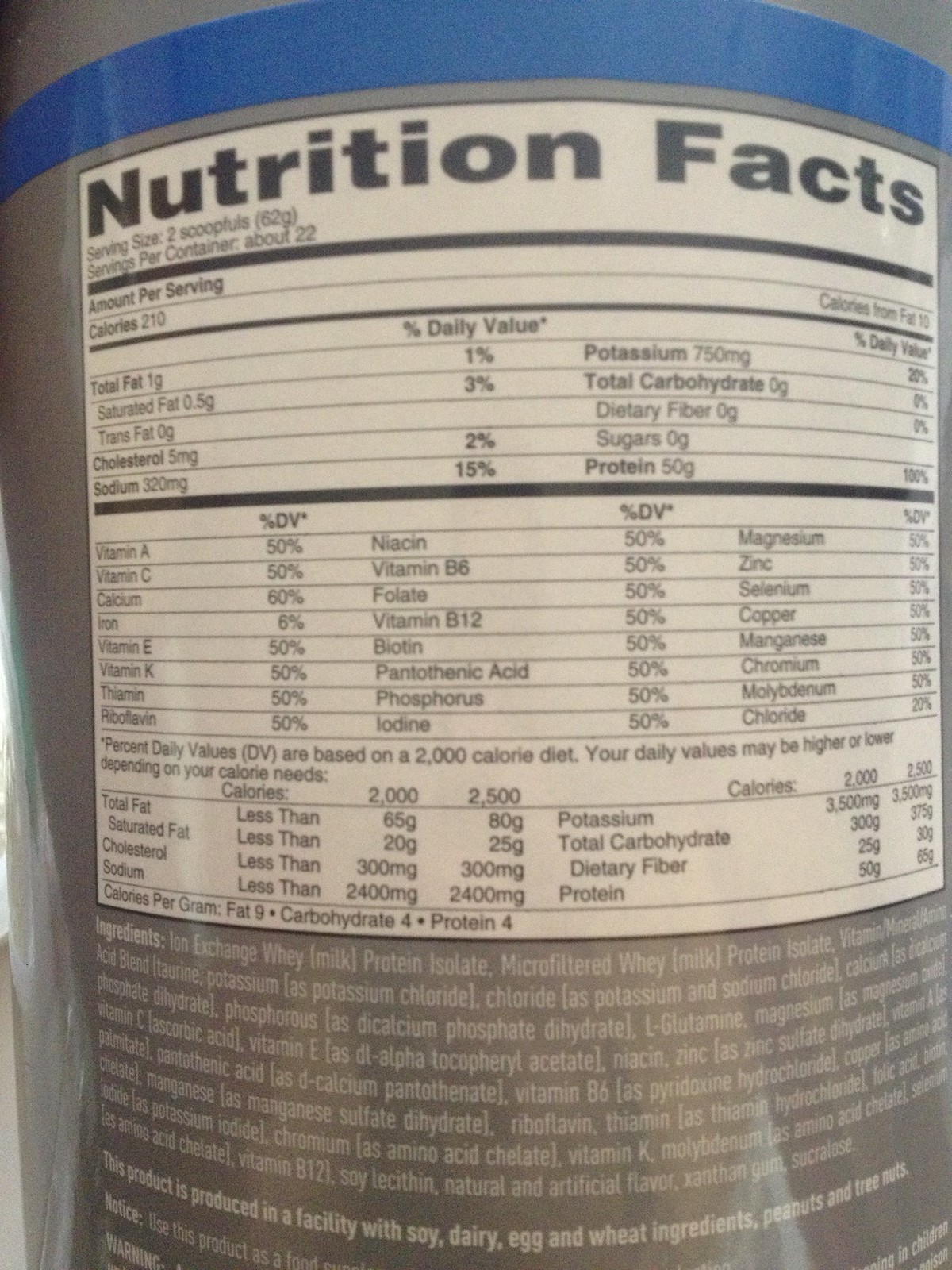The image is a detailed, close-up color photograph of the Nutrition Facts label on the backside of a gray, cylindrical container with a blue stripe near the top. The label entirely fills the frame and displays large, prominent black text reading "Nutrition Facts" at the top of a white box. Below this heading, the serving size is specified as "two scoopfuls" (62g), and the container is said to contain approximately 22 servings. The list of nutritional information includes values for calories, total fat, saturated and trans fat, cholesterol, and sodium, each with the daily value percentages listed to the right. The label also details various vitamins and minerals in three vertical columns. Beneath the Nutrition Facts, in white text on a gray background, the ingredients are listed, starting with "Iron Exchange Whey (Milk Protein Isolate)." Additional notices, warnings, allergens, and other information are present below the ingredients. Light shines on the can from the left side, creating visible reflections on its front.